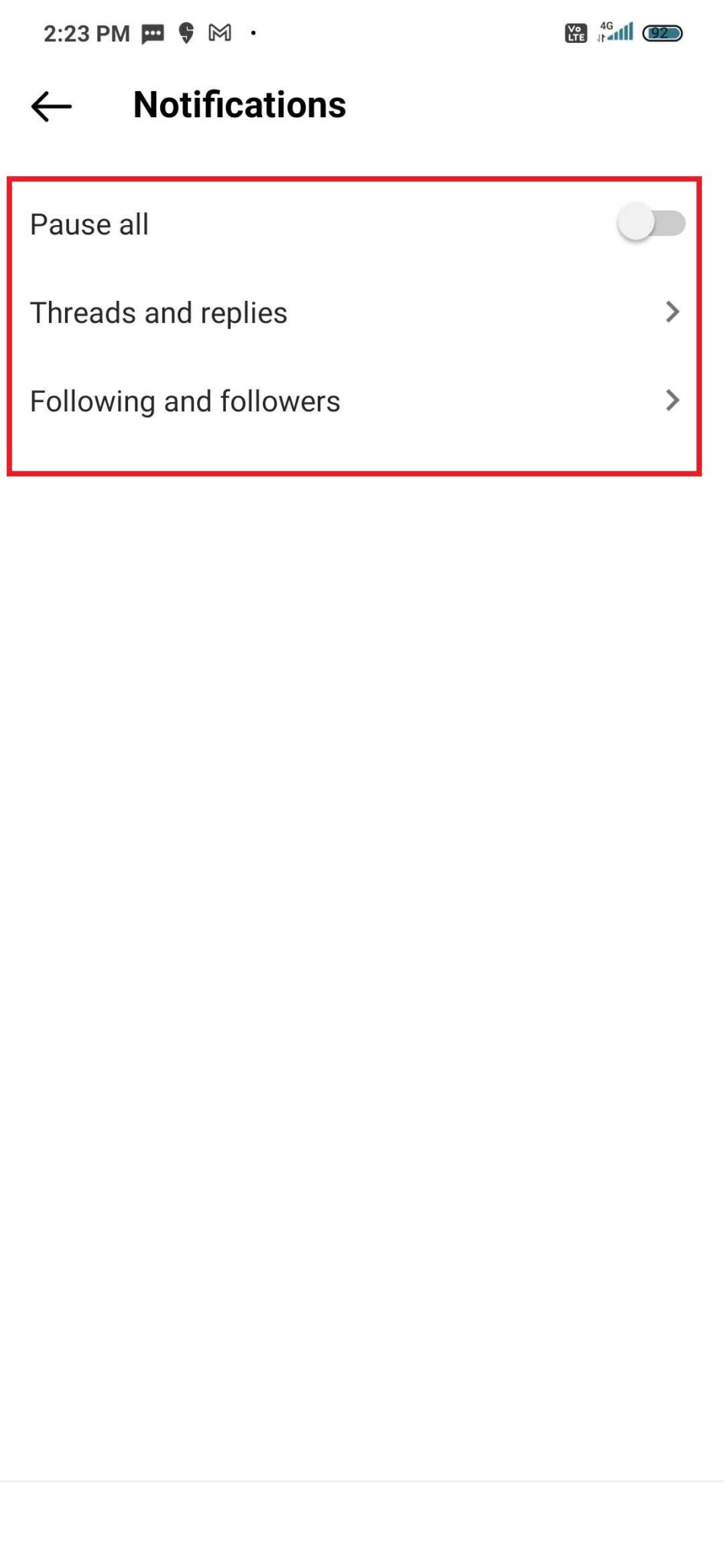The image features a white background, prominently displaying the time "2:23 p.m.". There is an arrow icon, likely indicating notifications, and a red rectangle that highlights specific information on the screen. The user interface shows a "Pause All" option which is currently turned off, accompanied by a "Taco Bar" section. Additionally, there are sections labeled "Threads" and "Replies", each marked with a right-facing arrow. Below these sections, the screen also shows "Following" and "Followers," also with right arrows for navigation.